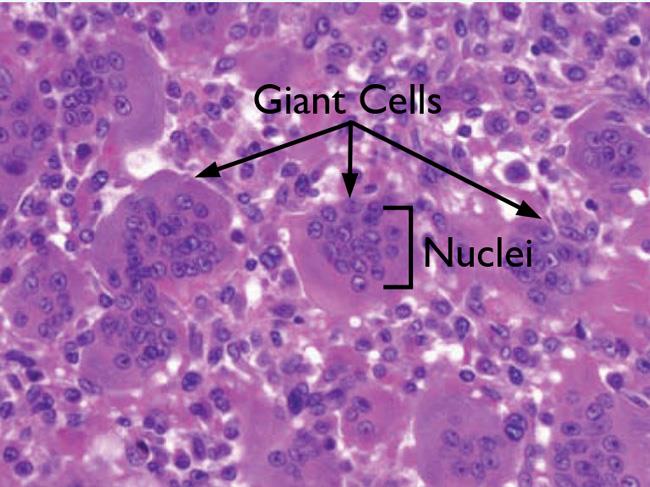The image depicts a microscopic view of numerous cells, predominantly colored in shades of lavender, darker purple, and reddish-purple, with white areas interspersed between the cells. Central to the image is the label "giant cells," which three arrows designate toward larger circles containing many smaller, uniquely circular cells. Additionally, a bracket below these larger cells highlights the term "nuclei," emphasizing the clusters of tiny, round cells within. The detailed scientific labeling and the intricate coloration suggest that this image is likely intended for educational purposes in a science textbook, showcasing the detailed structure and classification of cellular components under a microscope.